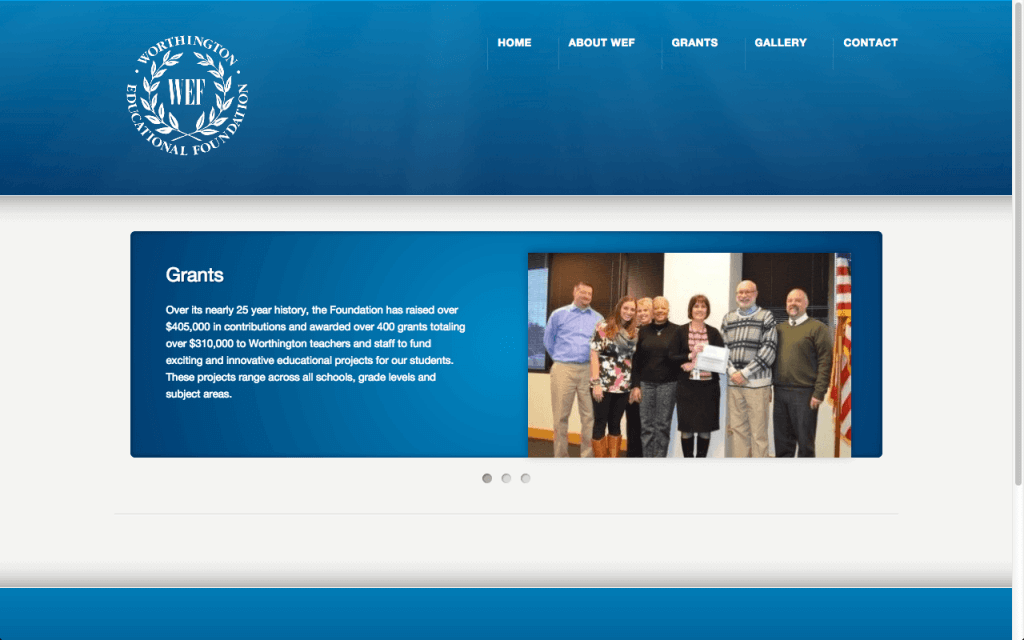This image showcases the Worthington Educational Foundation's website. Central to the design is the organization's emblem, a white badge featuring the initials "WF," surrounded by a laurel wreath, and encircled by the words "Worthington Educational Foundation." 

At the top of the webpage are four navigation tabs labeled "Home," "About WF," "Grants," "Gallery," and "Contact," all presented in a clean, white font against a blue background. In the main content section, a blue backdrop supports a detailed explanation of the grants offered by the foundation.

On the right side of the blue section, an image displays seven individuals of light-skin tones, dressed in business attire suitable for an office environment, standing together. Below this photograph, the text in white reads: "Grants. Over its nearly 25-year history, the foundation has raised over $450,000 in contributions and has awarded over 400 grants totaling over $310,000 to Worthington teachers and staff to fund exciting and innovative educational projects for our students. These projects range across all schools, grade levels, and subject areas." The paragraph concludes with an ellipsis, suggesting additional information follows.

At the bottom of the screen, a blue bar appears, and along the right edge, a scrollbar is visible, indicating that more content lies below the initial viewable area.